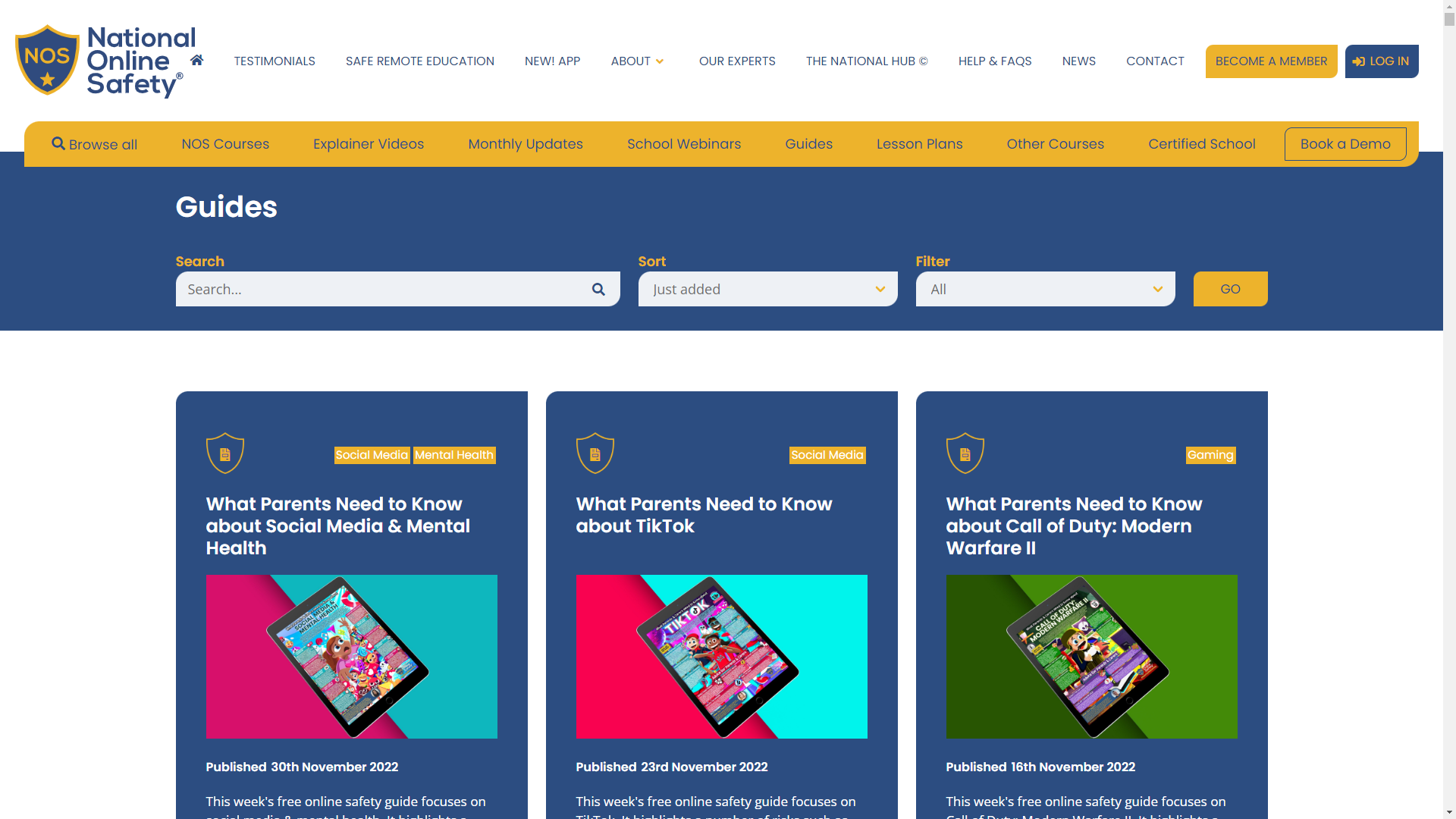This image is an advertisement for the National Online Safety website, showcasing a detailed and user-friendly interface. The top menu bar contains various tabs organized from right to left: Testimonials, Safe Remote Education, New App, About Our Experts, National Hub, Help and Facts, News, and Contact. Adjacent to these tabs are two prominent rectangles—one yellow that reads "Become a Member" and another blue labeled "Log In."

Below the primary menu is a secondary navigation bar with additional tabs: "Browse All" with a search icon, NOS Courses, Explainer Videos, Monthly Updates, School Webinars, Guides, Wisdom Plans, Other Courses, Certify School, and a 'Book a Demo' button.

Further down, the main content area is introduced by a blue square labeled "Guides," accompanied by a set of search and filter tools. These tools include a search bar with a magnifying glass icon, a dropdown menu for sorting, a filter menu set to "All," and a "Go" button.

The visible content features three article previews, each displayed in individual boxes. These articles cover various aspects of social media, with one specifically focused on gaming.